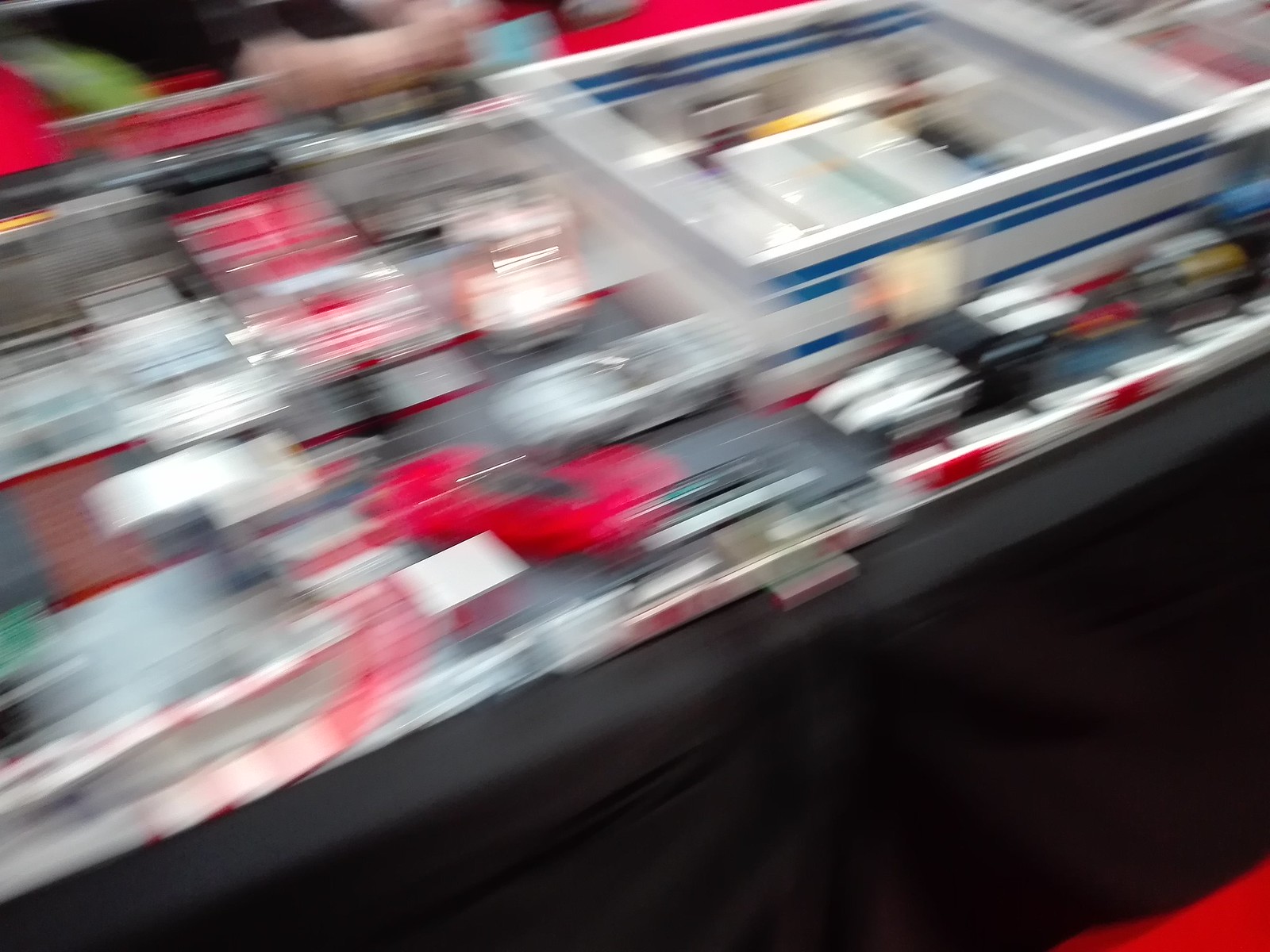This is an extremely blurry photograph of a diorama set up on a black table with a black tablecloth. It appears that the image was captured while the camera was in motion, contributing to the streaky colors and lack of clarity. The diorama features a LEGO-type layout with a small white and blue-striped building, roughly four LEGO pieces high, situated to the right. In front of this building are multiple model cars, including a red sports-like Ferrari, a white Porsche-like car, and a silver Porsche-like car, all oriented towards the left of the image. While the color red is prominent in the scene, giving hints of additional details, the lack of focus makes it challenging to discern specific objects accurately. A person's arm, clad in a black short-sleeve shirt, is faintly visible at the top of the image, but their face is not in view. The overall composition suggests a hobbyist's display, possibly of model cars on a LEGO roadway, atop a black-clothed table above red carpeting.